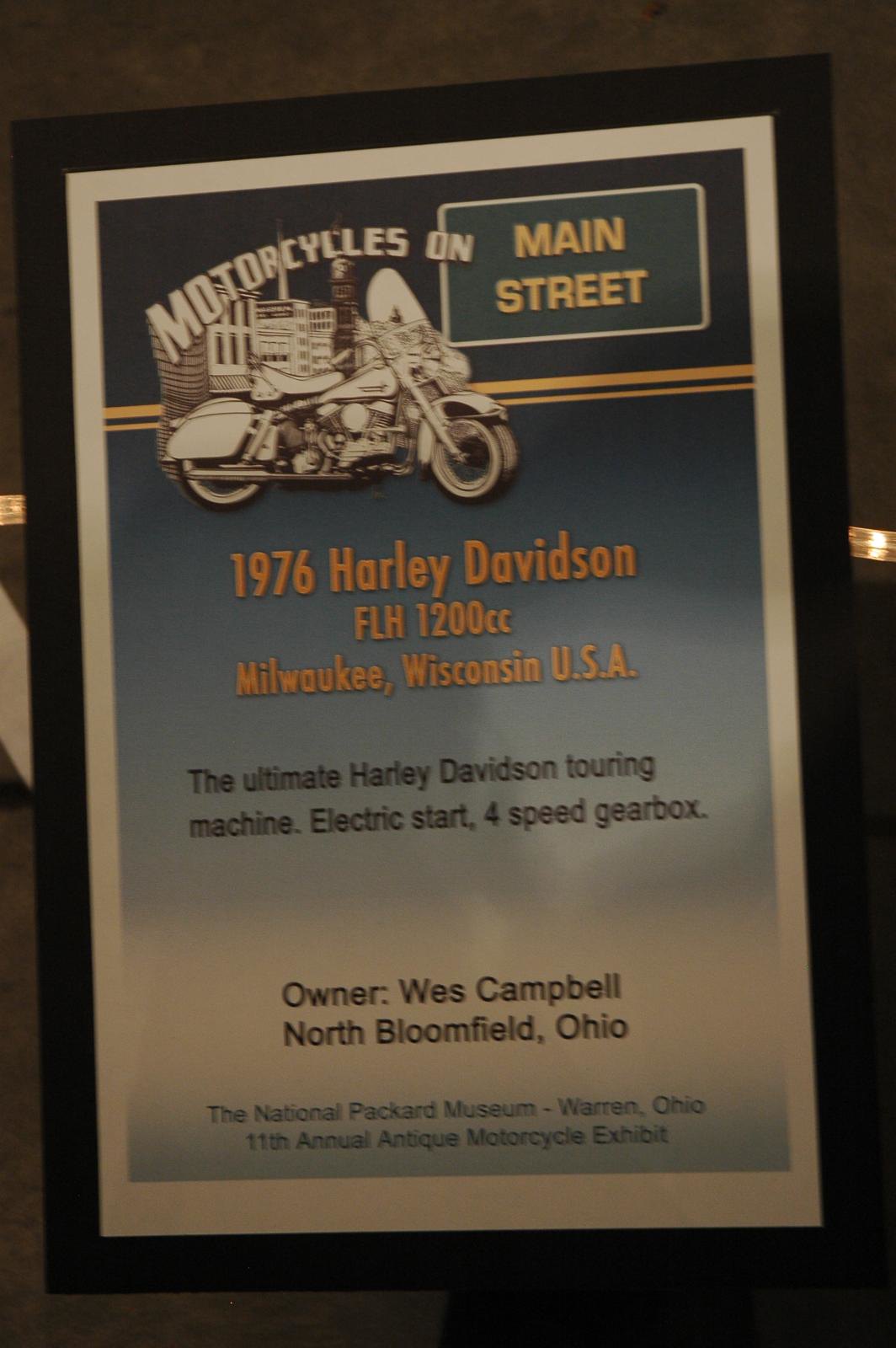The promotional poster is elegantly framed in a black frame and mounted on a gray wall with gold trim. The poster features a detailed black and white drawing of a motorcycle in the top left corner, set against a gradient blue background that transitions to white towards the bottom. In white text, "Motorcycles On" is prominently displayed, followed by a green rectangle with a white border and yellow font that reads "Main Street." Below the motorcycle drawing, orange text announces "1976 Harley-Davidson FLH 1200cc Milwaukee, Wisconsin, USA." Beneath this, black text describes it as "The Ultimate Harley-Davidson Touring Machine," featuring an "Electric Start," a "4-Speed Gearbox," and identifying the owner as "Wes Campbell, North Bloomfield, Ohio." At the bottom, the poster details the event as being held at "The National Packard Museum, Warren, Ohio," for their "11th Annual Antique Motorcycle Exhibit."